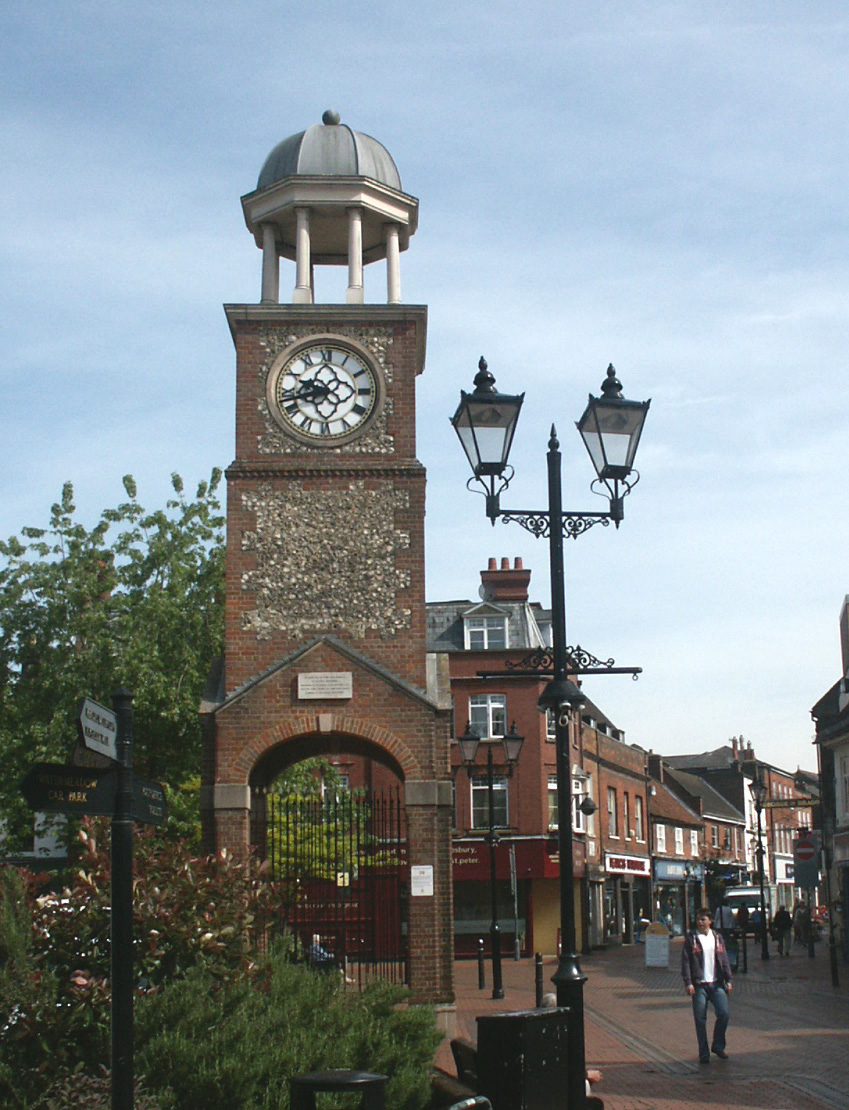The image depicts a picturesque town square with a prominent, red-bricked European-style clock tower. The clock tower features intricate small stonework in the middle and a black wrought iron gate, roughly 20 feet tall, at its base, possibly guarding a protected area. The clock face is white with black Roman numerals and hands, showing the time as 9:43, likely in the morning. Atop the tower is a striking rotunda adorned with a green roof. The scene is set under blue skies with a few wispy white clouds, perhaps indicating a slightly overcast condition.

In the foreground, there is a tall lamppost and a signpost directing towards an off-screen park. A couple of bushes and a large tree frame the left side of the tower, while various buildings line the winding street that trails off to the right in the background. Scattered pedestrians stroll along the street, which is lined with shops and dotted with an abundance of green vegetation. The town square exudes a serene morning atmosphere, with its harmonious blend of earthy brick tones, vibrant greenery, and the subtle gray-blue sky.